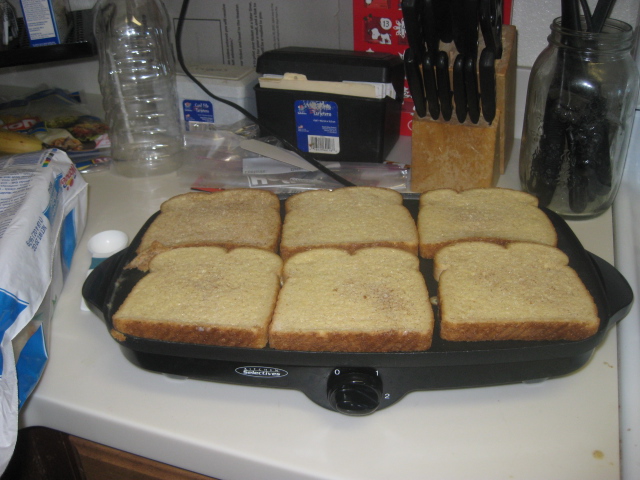The image showcases a bustling kitchen scene centered around a griddle located prominently on a white counter, where six slices of French toast are sizzling, the buttered sides facing up and ready to be flipped. The griddle knob is set to level two, hinting that they are mid-cook. Surrounding the griddle, an open loaf of bread rests to the side, partially out of frame. In the background, a variety of kitchen essentials are scattered: a gallon-sized mason jar filled with an assortment of kitchen utensils, a fully stocked wooden knife block with black-handled knives, and an emptied plastic bottle, possibly previously containing water or juice, which is segmented and bumpy. An assortment of other items, including storage bags, a black plastic recipe box with dividers, and a red kitchen towel, add to the organized chaos. A banana can also be spotted amidst the countertop clutter. The overall focus remains on the preparation of what appears to be a delicious batch of French toast.